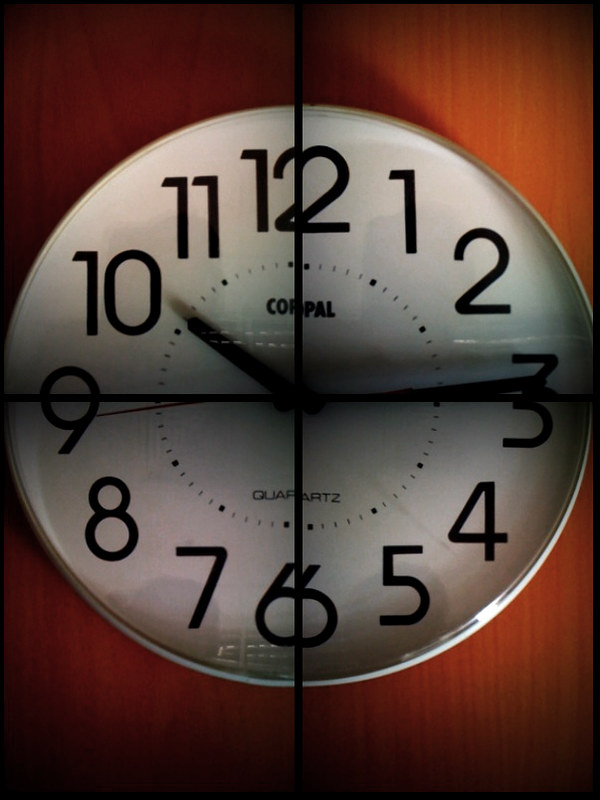This detailed photograph captures a retro-style wall clock affixed to a reddish-brown wooden paneled wall, likely cherry wood, displaying its grain texture prominently. The clock has a pure white face with large, black, retro-looking numerals from 1 to 12. The center of the clock sports additional markings and features two words: "CUPPAL" and "QUARTZ" just below it. The clock is enclosed in glass, adding a slight sheen over its surface. Notably, a dark black rectangular line vertically splits the clock in two, disrupting the numbers 12, 6, and forming a double effect, almost creating a double 2 and double 6. There is also a horizontal line, creating a black cross that divides the clock into four quarters. The hands of the clock, including the second hand, are slightly blurred, indicating the current time as 3:50. Shadows cast over the clock face and some minor stains suggest it is a slightly older model.